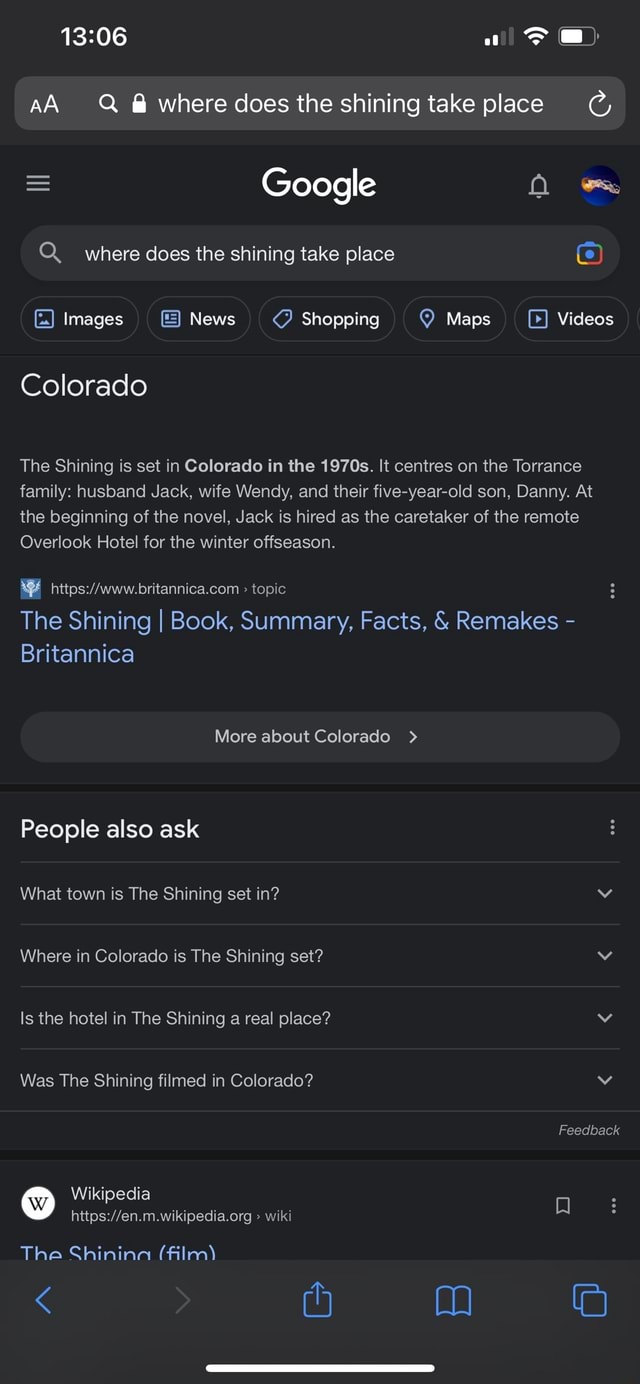The image depicts the homepage of the Google website with a search query in progress. At the top center of the webpage, there is a prominent and clean Google search bar, just below which the colorful Google logo is situated, occupying the center of the screen. On the left-hand side, a menu icon, represented by three horizontal lines, is visible. To the right-hand side, the user’s profile picture and an adjacent icon indicating notifications or additional menu options are present.

In the main search bar, the user has typed "where does The Shining take place." Below the search bar, several buttons offer different options for exploring the search results, including images, news, shopping, maps, and videos. Among the search results, a snippet provides a succinct answer: "Colorado." Following this, a brief summary elaborates, explaining that "The Shining" is set in Colorado during the 1970s and follows the Torrance family—husband Jack, wife Wendy, and their five-year-old son Danny. It mentions that Jack is hired as the caretaker of the remote Overlook Hotel for the winter off-season.

Further, there is a hyperlink to Pertanica's website, titled "The Shining: Book Summary, Facts, and Remakes," shown in blue and clickable. Below this, a long oval button invites users to learn more about Colorado. Further down, a "People also ask" section appears, with a question regarding the specific town setting of "The Shining," which can be expanded via a drop-down option. Next to this section, three dots provide additional menu options for that particular question.